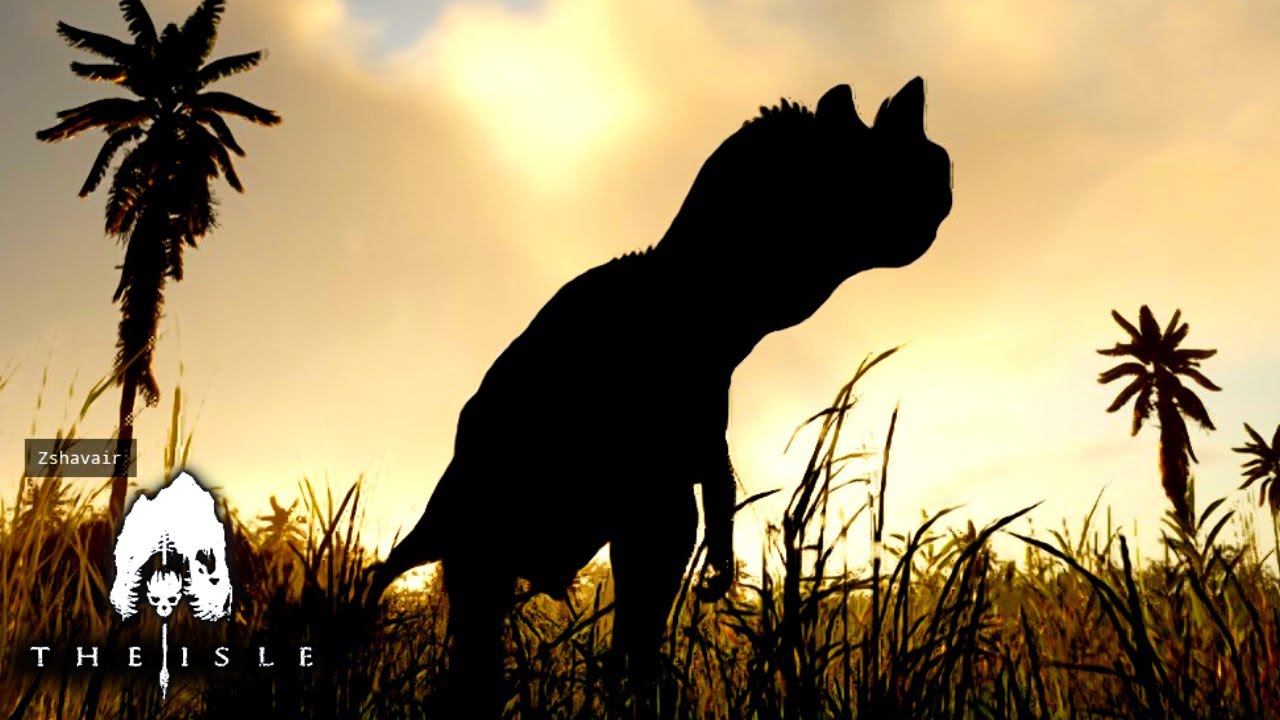The image depicts a dramatic scene from a video game, likely "The Isle," showcasing an orange sunset or sunrise with a dinosaur prominently featured in the foreground. The dinosaur, which resembles a T-Rex but with additional horns on its head, is captured in a black silhouette, standing on its hind legs amid tall grass. Surrounding the dinosaur are numerous ancient-looking palm trees, adding to the prehistoric ambiance. The sky above is predominantly covered with varying shades of clouds, though a small patch of blue is visible along with a brighter spot hinting at the sun behind. In the bottom left corner of the image, a semi-transparent gray rectangle features a logo with a white design depicting a skull on a pole, accompanied by the text "Z-S-H-A-V-A-I-R" and "The Isle."